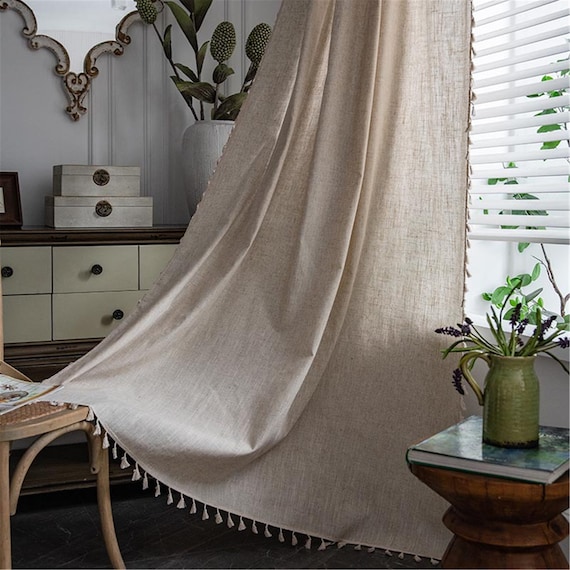In this daytime photograph of a bohemian-styled living room, the focal point is a beige, linen-like curtain bordered with small tassels, draped over a chair and seemingly held in place by a pamphlet or magazine. This curtain stretches from a window with white Roman blinds, adding to the neutral color palette. To the left of the curtain, there's a potted cactus placed near an ornate mirror on the wall, while two cream boxes rest on top of a sideboard featuring yellow drawers with small brown handles. On the right side of the curtain, a green iridescent jug filled with lavender plants sits on a coffee table book on a small wooden nightstand. The sunlight streaming through the window illuminates the room, highlighting the bohemian decor and creating a warm, inviting atmosphere.